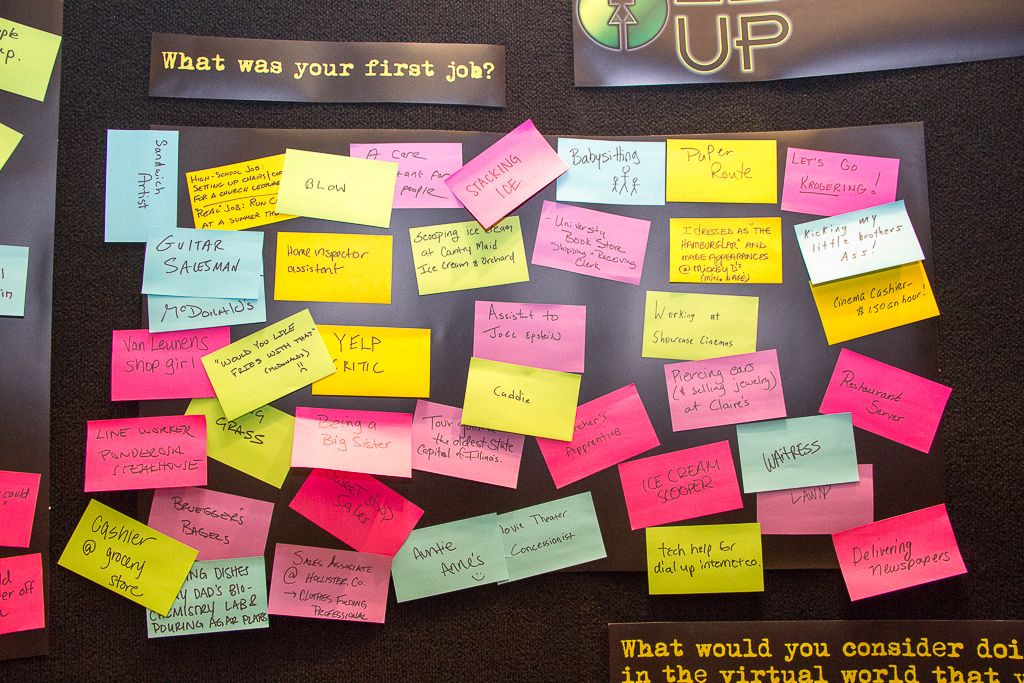The image depicts a black bulletin board affixed to a black wall, displaying a prominent written question at the top: "What was your first job?" Below the question, numerous colorful post-it notes—ranging in shades from blue and yellow to green, hot pink, purple, and light pink—are scattered across the board. These notes contain various hand-written responses detailing individuals' first jobs. Some of the legible answers include "Waitress," "Guitar Salesman," and "Cashier at a Grocery Store." The setting appears to be indoors, and further down in the bottom right corner, partially obscured text reads, "What would you consider doing in the virtual world," indicating an additional prompt.